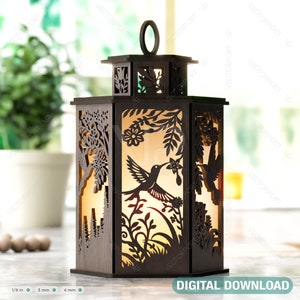This detailed close-up photograph captures a beautifully crafted bronze decorative lantern, ideal for an outdoor setting like a picnic table. The lantern, designed in a hexagonal shape with six intricately engraved panels, is predominantly made of metal housed within a dark brown wooden frame. Its larger base tapers to a smaller top, adorned with a ring for hanging. The front and central panels vividly depict nature-inspired scenes: a hummingbird with outstretched wings drinks from a star-shaped flower amidst detailed foliage, while another bird appears to be in flight toward pine cones on deciduous and evergreen branches. The carvings reveal silhouettes of various flora, including leaves, stems, and flowers, meticulously rendered against the contrasting light brown or orange accents where the wood has been carved away. The lantern sits on a marble countertop, flanked by scattered wooden circular beads and a white ceramic pot brimming with dark green herbs. Sunlight streams through windows in the background, emphasizing the daytime setting. In the bottom right corner, a blue screen rectangle features the text "DIGITAL DOWNLOAD" in white capital letters.